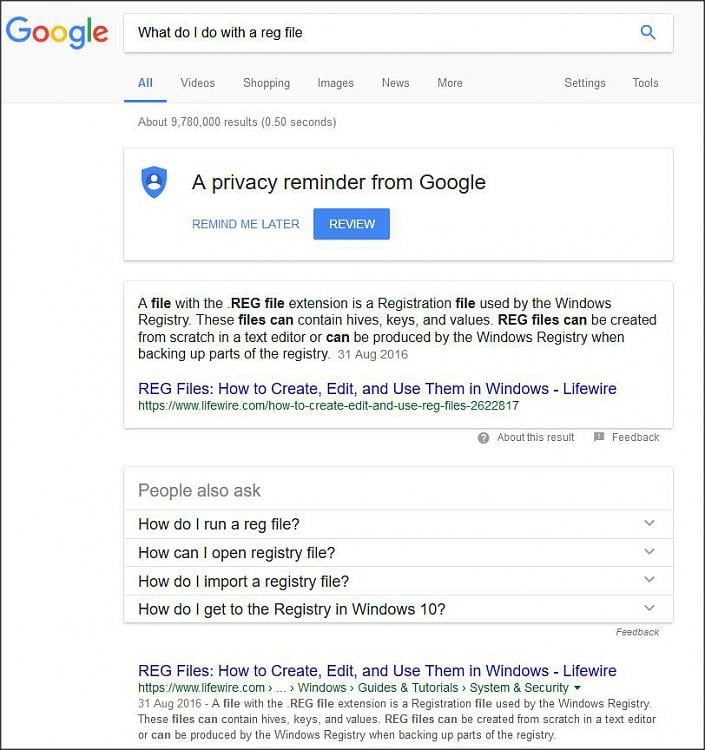A screenshot displaying a Google search results page with the query "what do I do with the reg file?" highlighted in the search box. The interface shows the standard Google tabs for "All," "Videos," "Shopping," "Images," "News," "More," "Settings," and "Tools," all underlined in blue. Below the search bar, it indicates approximately 9,780,000 results retrieved in 0.50 seconds. Additionally, there is a "Prophecy Reminder" from Google with options to "Remind me later" and "Review," where "Review" is written in white on a blue rectangular button.

In the search results, a description explains that a .reg file is a registration file used by the Windows Registry and may contain hives, keys, and values. It mentions that these files can be created in a text editor or by the Windows Registry during a backup. One of the search results is titled "Reg files, how to create, edit and use them in Windows," dated August 31, 2016, and appears multiple times, emphasizing its relevance to the query.